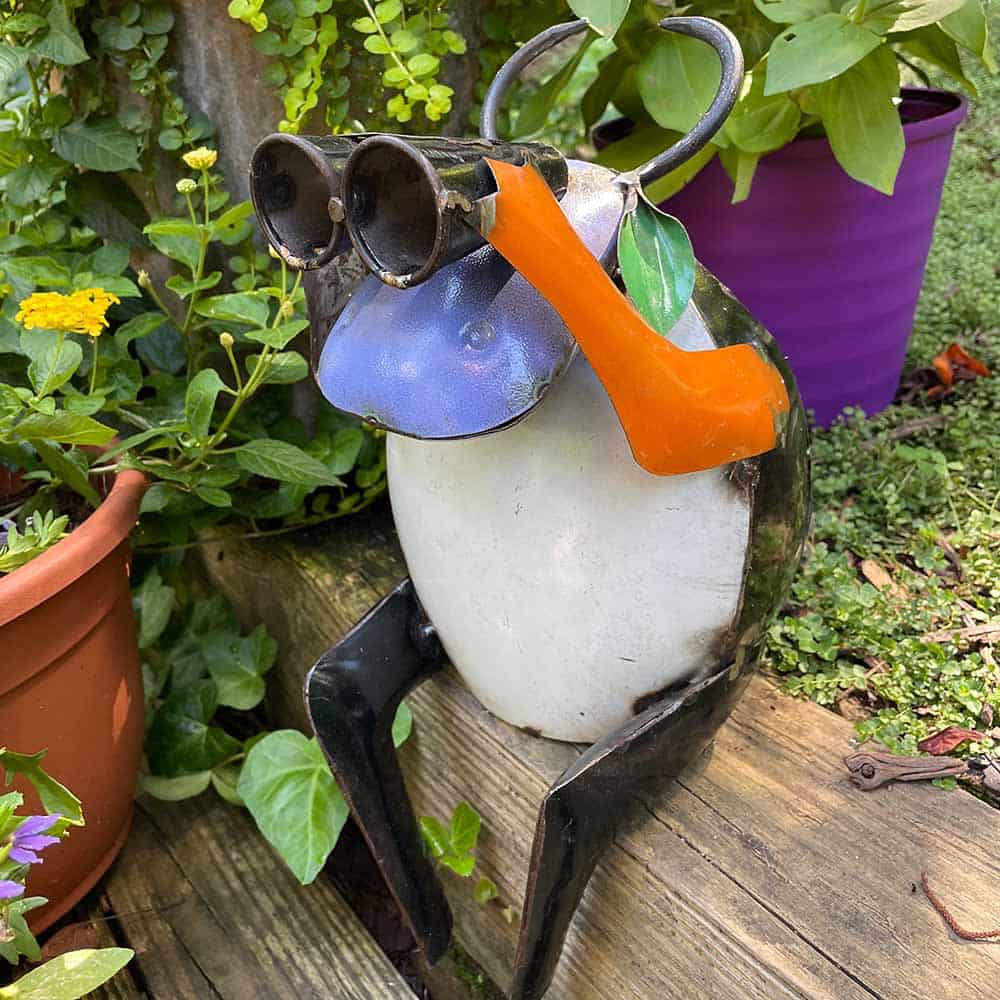This image captures a meticulously arranged multi-level garden. Each tier is supported by weathered wooden planks, hosting a variety of plants. The uppermost level features a plant situated next to a striking purple-painted terracotta pot on the top right. On the lower left, a typical terracotta pot blooms with yellow flowers, adding a pop of color. The centerpiece of the garden is a quirky decor item crafted from recycled metal. This imaginative creature, resembling a whimsical blend of a cow and frog, boasts a black body with a white stomach. It holds a pair of black binoculars with its orange arm. The creature's design is further enhanced by its purple bill, black horns, and a green ear, giving it a playful yet intriguing character as it appears to watch over the garden through its binoculars. The vibrant colors and eclectic features of this decor item imbue the garden with a sense of fanciful charm.